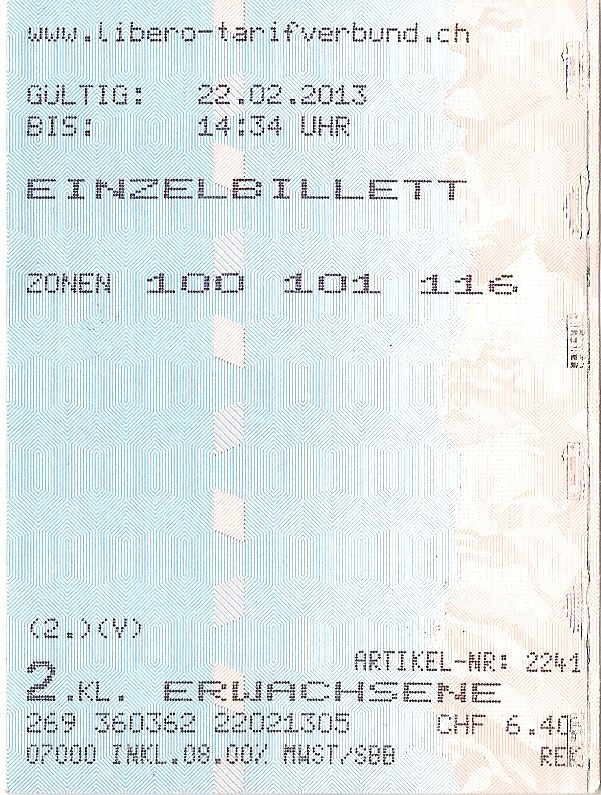The image is of a ticket or receipt predominantly featuring text in a foreign language. The ticket has a colorful design with sections in pink and blue on the left and light greenish and purplish hues on the right. At the top of the ticket, it reads "www.librero-tarifverbun.ch," followed by several key details: "GULTIG: 22.02.2013" and "BIS: 14:34 UHR." Below these, in large black letters, the word "EINZELBILLETT" is displayed, followed by "ZONEN 100 101 116." Toward the bottom of the ticket, more text appears in large black letters: "2.KL. ERWACHSENE." Additional numbers are scattered throughout the lower section, including 269, 360, 362, 220, 213, and "CHF 6.40" near the bottom right corner, with "REC" noted beneath it. Overall, the ticket appears fresh and new, marked by a mix of bold numbers and alphabetic characters in various sizes and styles.